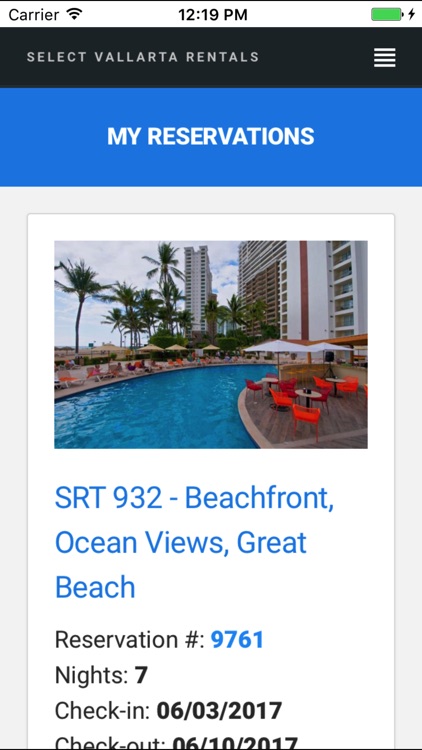Screen capture of a smartphone displaying either an app or a webpage. The top-right corner shows a lightning bolt logo and a fully green battery charging symbol. The time reads 12:19 p.m. In the top-left corner, "Carrier" is displayed next to a full Wi-Fi connection symbol. Below, a dark banner reads "Select Valarta Rentals" with a four-line drop-down menu icon in the top-right corner. 

Below this is a blue banner with white text stating "My Reservations." The main section features an image of a hotel or resort with a swimming pool. The backdrop shows a white high-rise hotel or resort, surrounded by pool chairs and umbrellas. Beneath the image, blue text reads "SRT 932 Beachfront, Ocean Views, Great Beach." Additional details include: 

- Reservation Number: 9761
- Nights: 7
- Check-in: 06-03-2017
- Check-out: 06-10-2017.